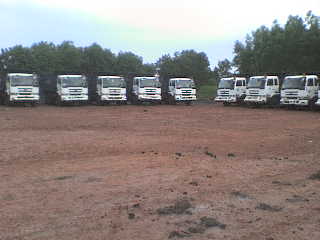This is a photograph depicting a collection of trucks parked in an outdoor setting, likely from the 1980s or 1990s. The scene is a large, empty lot covered in brown dirt or dry grass, with some large piles of dirt scattered around. The trucks are arranged in two rows forming an L-shape. One row of five trucks faces towards the viewer, while the other row of three trucks faces left. Behind the trucks, there are tall, fluffy green trees that frame the image. The sky above shows a light bluish-grey hue, gradually transitioning to white towards the top due to the light quality. Each truck appears to be white with a boxy shape and wide glass fronts, resembling semi-trucks or small commercial vehicles. The overall photo quality is low, making it difficult to discern finer details, and it has an older aesthetic.